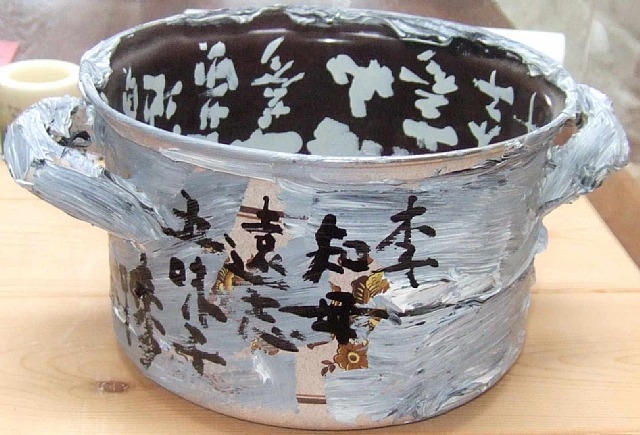This image captures a photograph of a two-handled ceramic pot, designed as an untitled work from 1978 by artist Nam June Paik. The pot, generously sized and evocative of a traditional soup pot, features a hand-painted exterior predominantly in white, created with thick and rough strokes. This base layer partly conceals an original floral design that peeks through in spots. Scattered across the white surface are black Asian symbols and letters, irregularly placed in a non-linear fashion. The pot's interior is painted in a contrasting black and showcases similar white Asian writing. The crafted piece sits on a light brown hardwood table in a real setting, with a candle observable in the background, emphasizing its authentic and functional artistry.